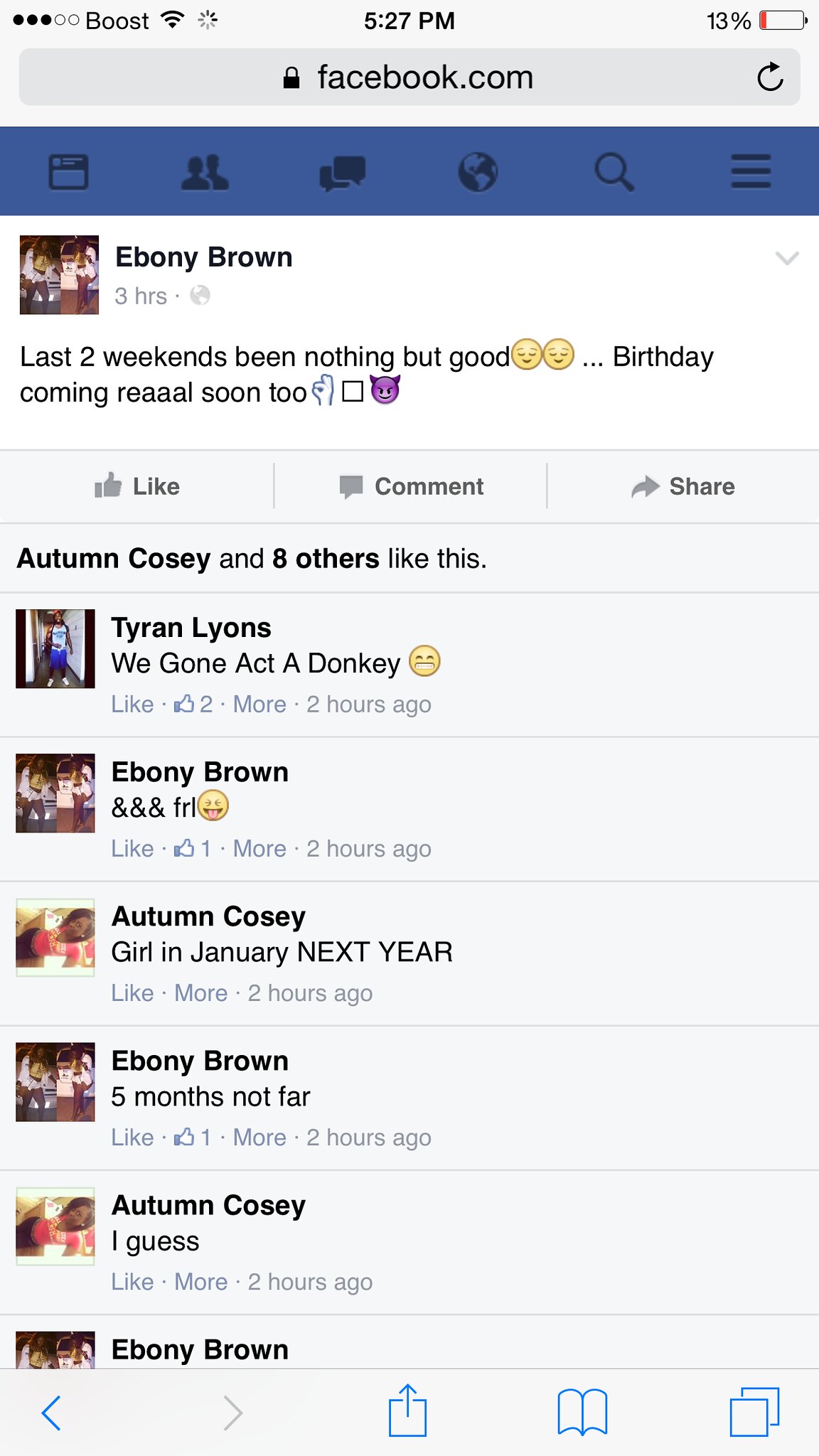This image is a screenshot of a Facebook page, captured on a phone screen with a battery level at 13%. The screenshot was taken using the Safari browser, as indicated by the icons at the bottom. At the top left of the screen, it says "Boost," and the time displayed is 5:27 PM. The web address bar shows "Facebook.com."

The post belongs to Ebony Brown and was posted three hours prior to the screenshot being taken. Ebony's status reads: "Last two weekends have been nothing but good 😊😊 Birthday coming real soon ✌️◻️😈." The empty square likely represents a failed emoji rendering.

The status received likes from Autumn Cozy and eight others. Tyronne Loins commented, "We gonna act a donkey 😁," to which Ebony Brown replied, "And and FRL 😛." Autumn Cozy commented, "Girl in January next year," and Ebony responded, "Five months not far." Autumn replied, "I guess," but Ebony's subsequent reply is cut off and not visible in the screenshot.

Next to each name in the comments section, there is a profile photo of the respective user.